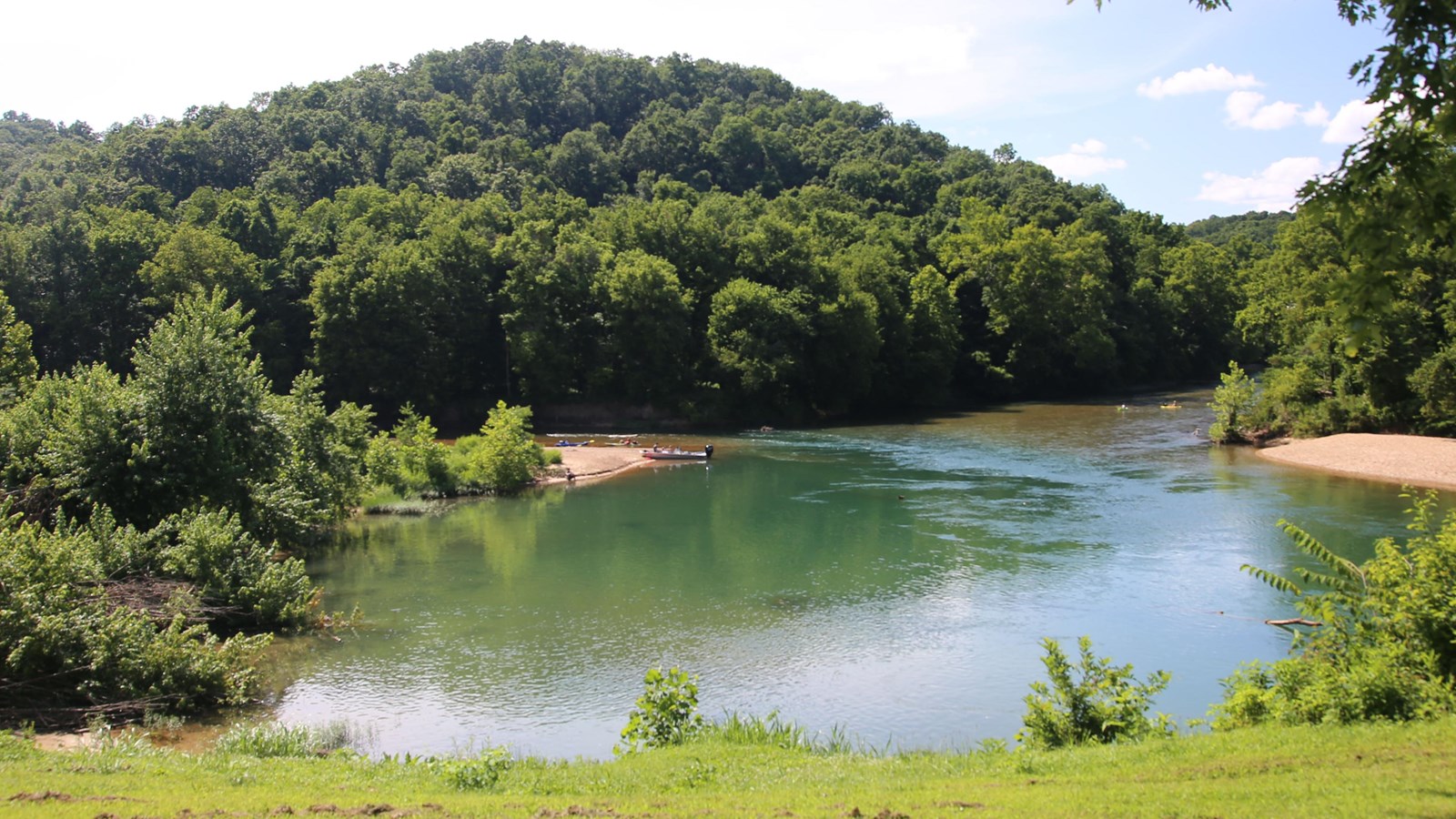The image is a color photograph taken on a bright, sunny summer afternoon, capturing a serene lakeside scene with a vivid blue sky at the top, occasionally dotted with white clouds in the distance. In the foreground, a lush, light green grassy field stretches out, dotted with smaller shrubs and bushes. The calm lake reflects the blue sky and the dense, vibrant green forest beyond it, creating a mirror-like effect. To the left, a shallow area is lined with extending bushes from the water's edge. On the right side, a sandbar is visible, with towering trees standing beyond it. At the center, a large, forested hill rises on the opposite shore, bathed in sunlight. Subtle ripples can be seen across the water’s surface, adding texture to the overall tranquility.